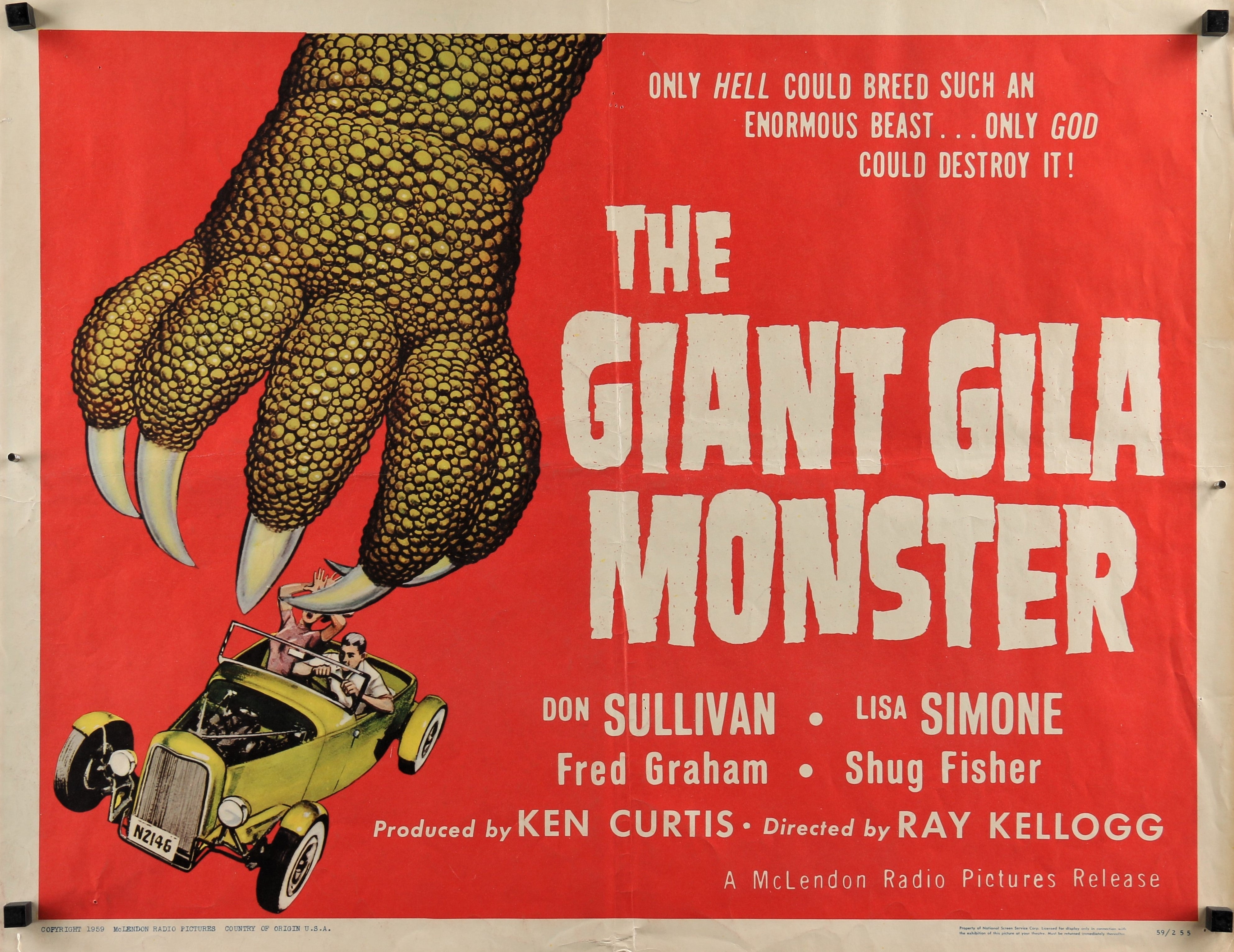This vibrant movie poster for "The Giant Gila Monster" features a dramatic red background with a bold white border. Dominating the scene, a gigantic, brownish-green dinosaur-like claw reaches menacingly towards a yellow antique car with the license plate N2146. Inside the car, a woman with a pink shirt can be seen screaming in terror, her hands raised in panic, while the focused husband at the wheel stretches his arms, seemingly ready to accelerate in a desperate bid to escape the monstrous threat. The harrowing tagline reads, "Only hell could breed such an enormous beast. Only God could destroy it." Prominent credits listed below the title include actors Don Sullivan, Lisa Simone, Fred Graham, and Shug Fisher, with the film produced by Ken Curtis, directed by Ray Kellogg, and released by McLendon Radio Pictures. The poster is further detailed with black tacks at each corner, suggesting it is pinned to a wall.